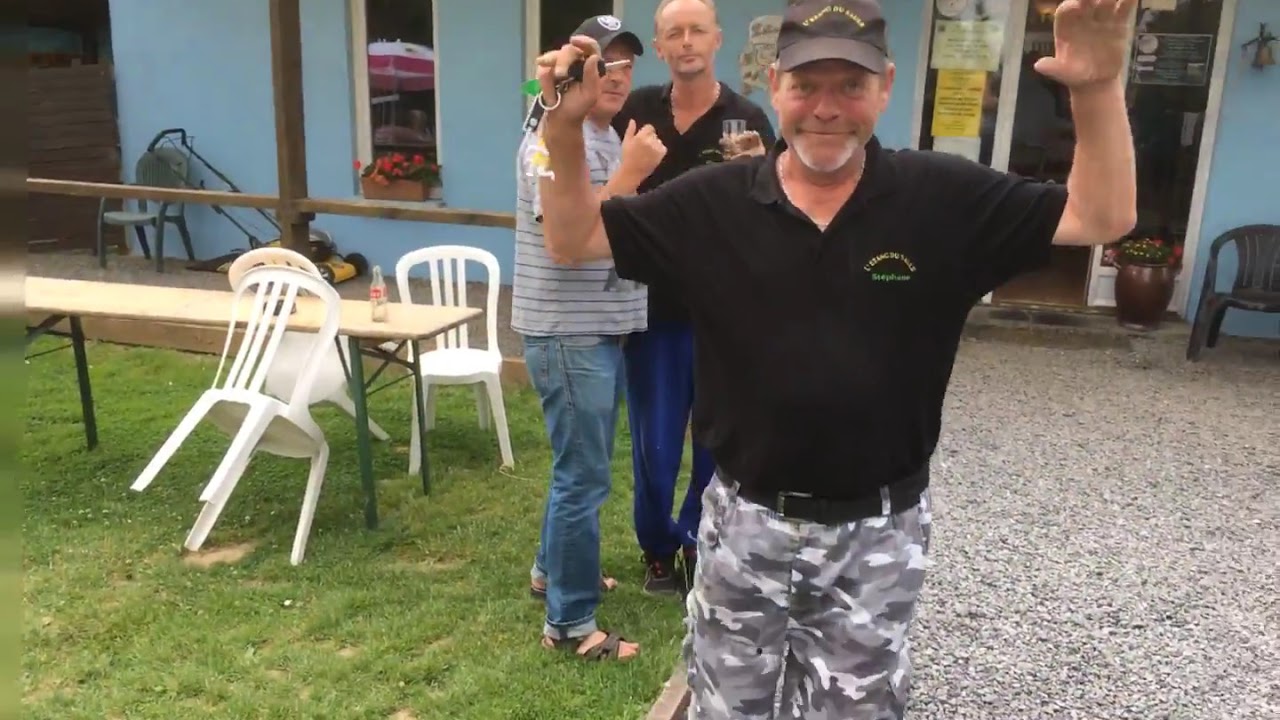In this detailed photo taken outside, a blue building with visible windows that resemble a country store forms the backdrop. To the left of the frame, there's a folding table with white plastic lawn chairs set up on a stone or gravel driveway. On the right side of the photo, three older white men are present. The man at the front, approximately 50 years old, sports a black baseball cap and a black polo shirt with a business logo on the chest. He also wears gray and white camouflage pants with a black belt. He is smiling and has his hands raised as if motioning "stop, don't shoot," holding keys in his right hand. Behind him, standing on a grassy area, are two other men. One is dressed in a gray striped shirt, blue jeans, and sandals, with a baseball cap, and the other wears a black polo shirt identical to the first man's, also displaying a business logo. Both men seem engaged in conversation. The setting suggests a casual, laid-back atmosphere with flower pots in the store's windows enhancing the scene.